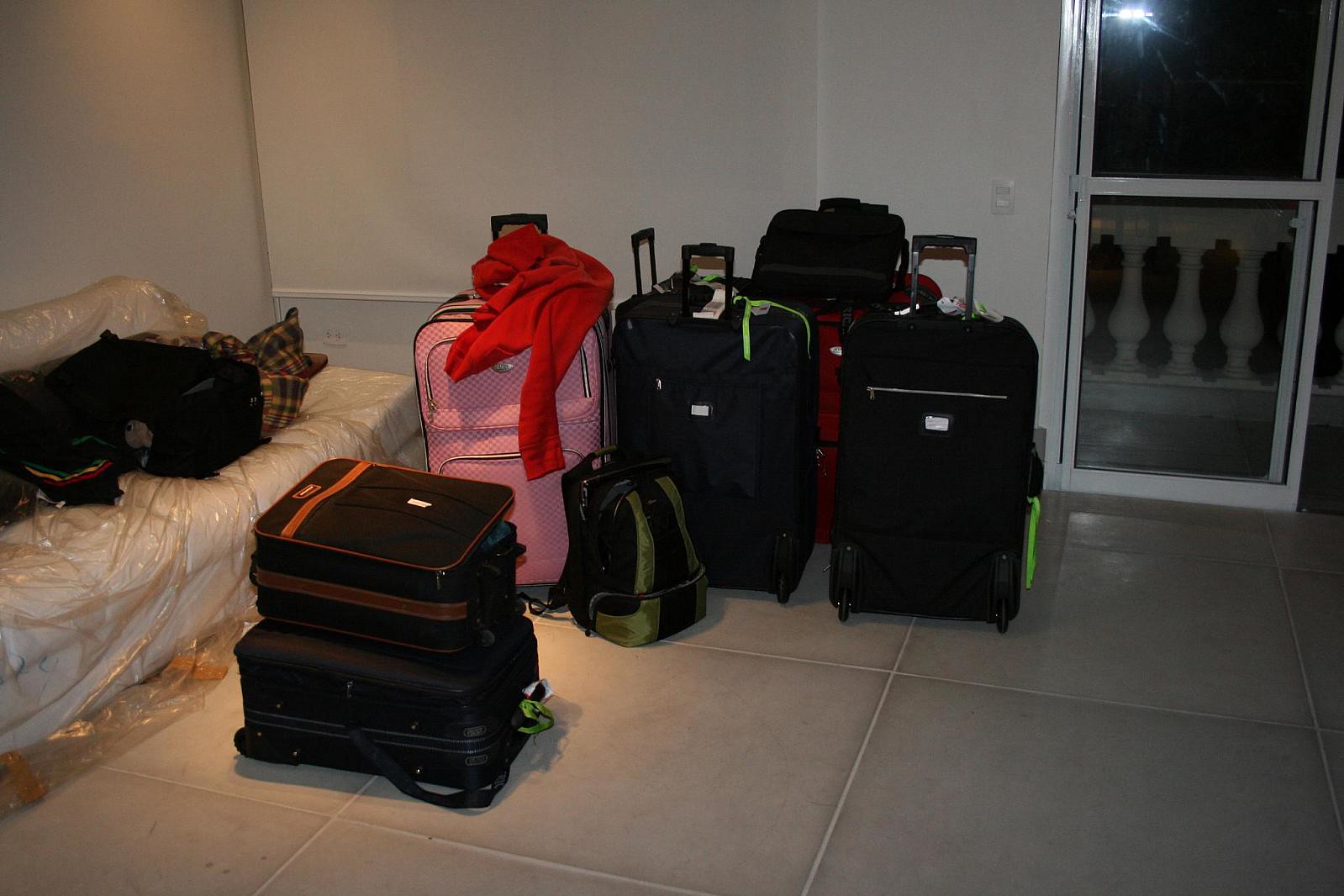This photograph captures a collection of luggage in what appears to be a hotel or rental room, characterized by its modern, minimalist decor. The floor is covered with large, light gray tiles approximately one yard square, and the walls are a clean, bright white. A white leather sofa, completely wrapped in clear plastic film, occupies the left side of the image, under a singular light fixture that softly illuminates the scene.

In the upper right corner, there's a glass sliding door, beyond which an ornate white stone balcony railing can be seen, indicating that it might be night outside as the camera flash is reflected in the glass. 

The luggage is varied and abundant, consisting of several rolling bags and backpacks. Prominently, there are two large black rolling bags situated front and center. Behind them stands a large red suitcase with a black laptop bag placed upon it. In the front, there’s a black and green backpack next to a striking pink rolling suitcase, with a red sweater casually draped over it. There are also two smaller black rolling bags stacked on top of each other in front of the larger suitcases. Additional pieces of black luggage are scattered, including one placed on the plastic-covered couch. 

This image conveys a moment of preparation or transition, with the neatly arranged luggage suggesting readiness for travel or a recent arrival.